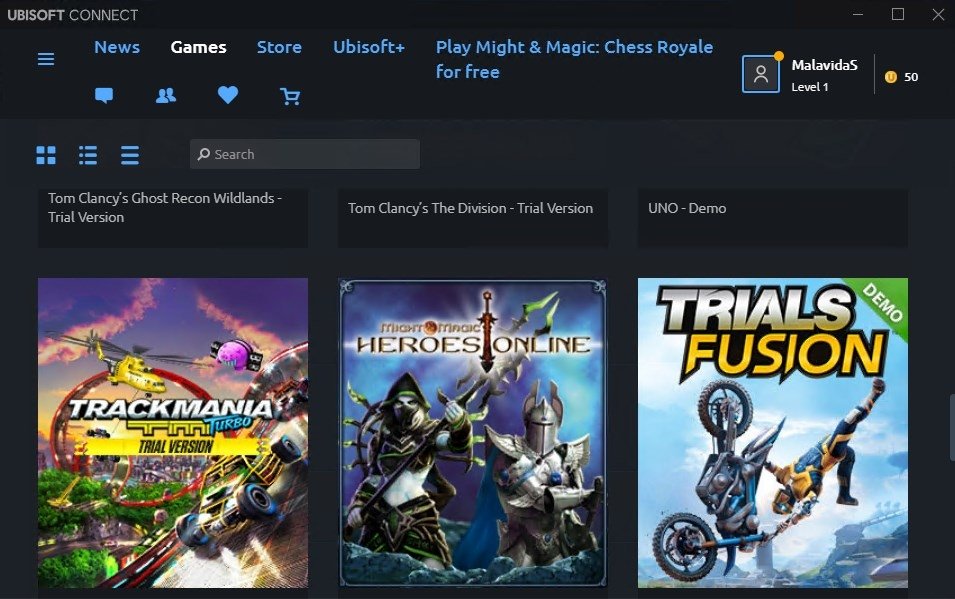The image displays the interface of Ubisoft Connect, a digital distribution platform by Ubisoft. In the upper right corner, there is an icon resembling a stick figure next to the username "Malavida S," indicating Level 1 status. To the right of the username, a yellow circle with the letter "U" in white prominently features the number 50. Below this, the following trial versions of games are listed: "Tom Clancy's Ghost Recon Wildlands," "Tom Clancy's The Division," and the demo for "UNO."

The main section of the interface showcases three game titles with corresponding images. The first image is of "Trackmania Turbo" trial version, depicting a car, a helicopter, and a circular track loop. The second image is for "Heroes Online," showing a knight in armor and a woman holding a spear. The third image features a dirt bike and a rider performing tricks, representing the "Trials Fusion" demo.